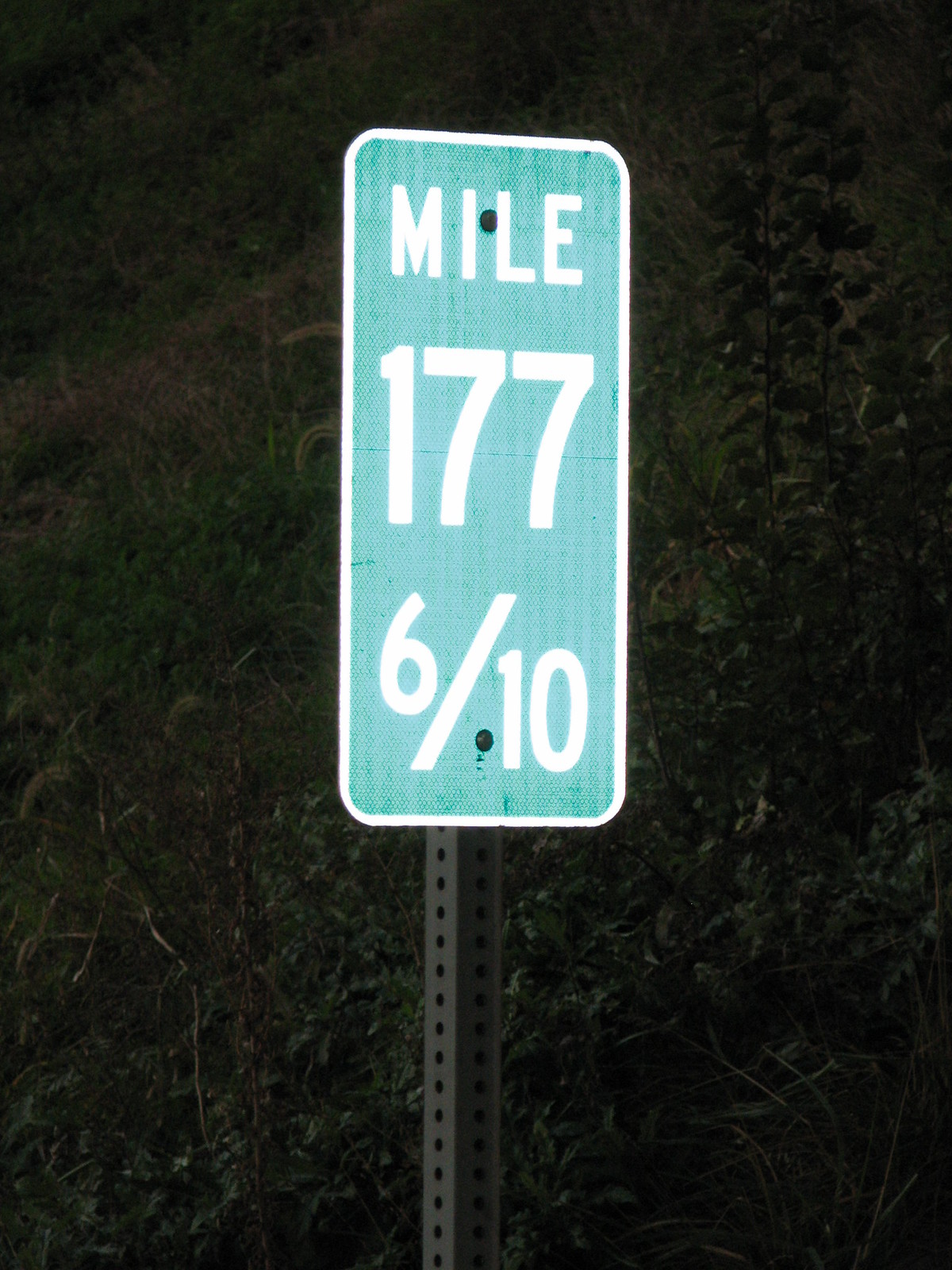The image features a vertically oriented, rectangular street sign with rounded corners. The sign is green with a white border and white text. The text reads "MILE" on the first line, "177" on the second line, and "6/10" on the third line, where the numbers are separated by a diagonal slash. This sign is affixed to a perforated, metal pole with evenly spaced holes running along its length. In the background, there is dense foliage from surrounding trees shrouded in darkness, suggesting that the photo was taken at night, likely with the aid of a flash to illuminate the sign prominently. The entire scene is composed in such a way that the green street sign attached to the metal pole is the clear focal point of the image.